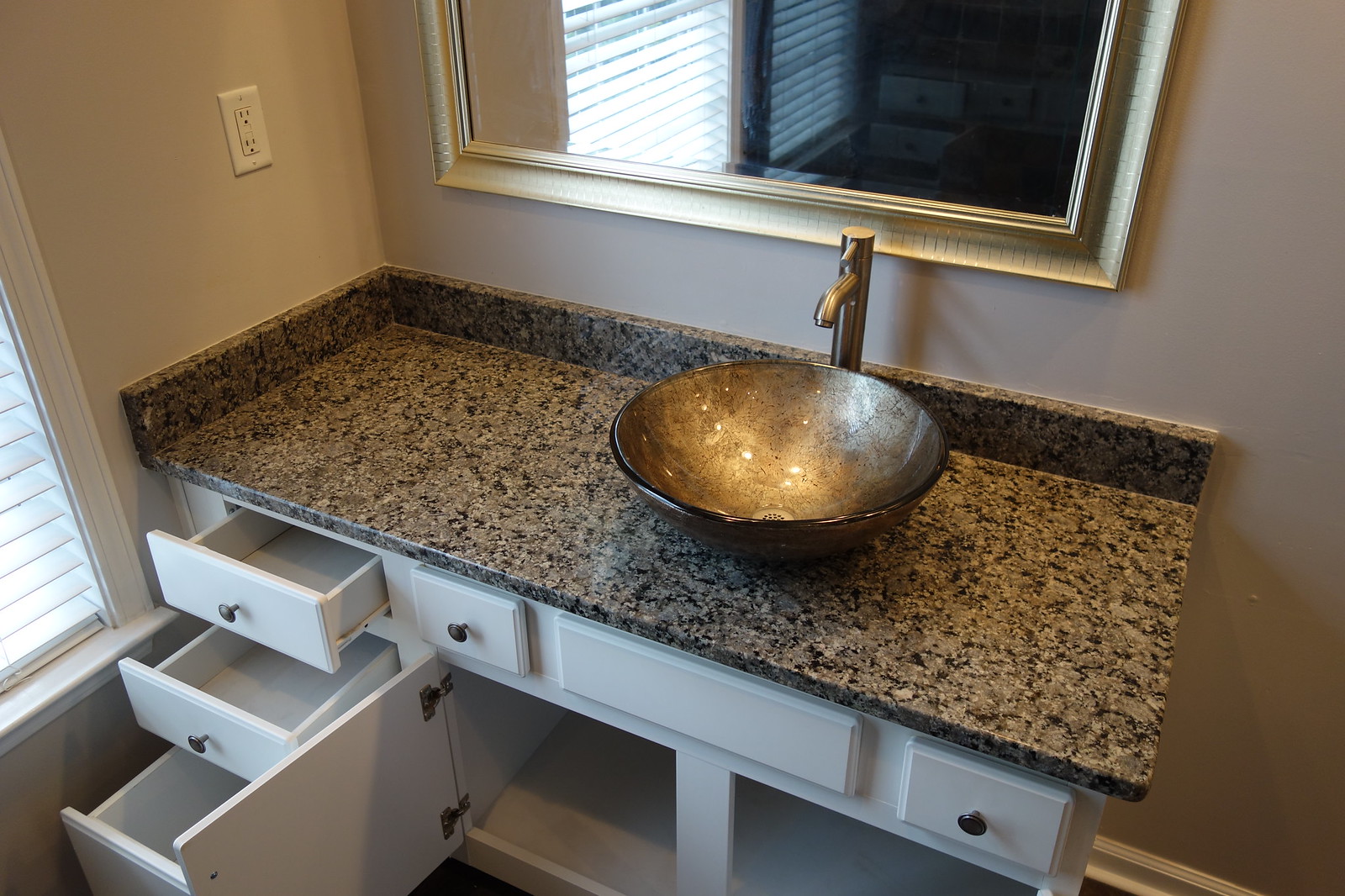This image showcases a modern bathroom with a striking countertop as the focal point. The countertop boasts a sophisticated marble design, predominantly featuring shades of black, gray, and hints of brown. The basin, integrated into the counter, exhibits a stone-like texture with a brownish tint and a glossy finish, enhancing its luxurious appearance.

The faucet is a standout feature with its contemporary design, consisting of a sleek, large pipe and a minimalist lever. This main pipe is complemented by a smaller pipe emerging over the basin, emphasizing its modern aesthetic.

Above the countertop, the walls are adorned in a warm brown hue, framing a mirror with an elegant golden frame. The mirror reflects the room’s further details, including windows and additional drawers. A dual-socket electrical outlet is visible on the wall, conveniently positioned for bathroom appliances.

The cabinetry below the countertop includes an array of drawers in stylish gray tones, equipped with sleek black handles. The drawers on the right are closed, offering a tidy storage solution, while several on the left are open, revealing ample space within.

Overall, the image captures the essence of a chic and well-designed bathroom space, blending modern elements with timeless finishes.